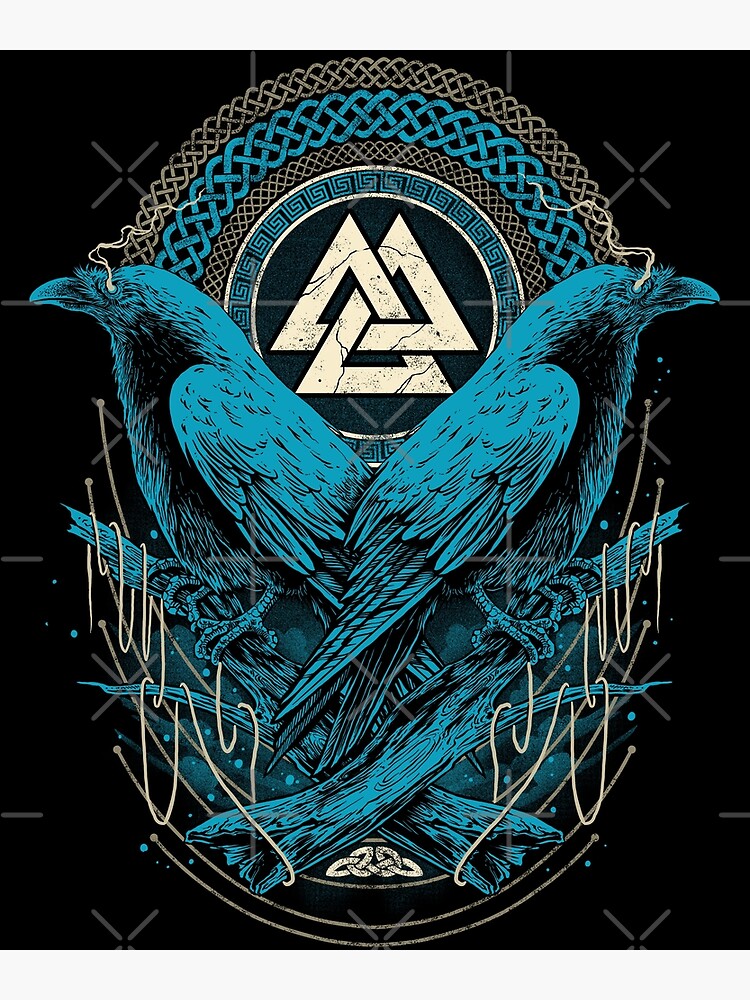This intricate drawing presents a captivating scene against a black backdrop, featuring two intersecting crows perched on blue branches. The crows, rendered in a striking blue or dark turquoise with hints of green and black under their wings, face opposite directions—one gazing left to right with its head pointed upward and the other from right to left. Their backs form a distinctive V-shape. Emerging from the eyes of each crow, white swirls trace a flowing path across the scene, looping around the branches and converging towards the bottom of the image.

Central to the composition, behind the crows, is a complex graphic consisting of three intertwined triangles, encompassed by successive bands of geometric patterns. The innermost band features intricate designs, followed by a blue patterned band and then a brown braided pattern. At the bottom of the image rests a prominent semicircle. Adding to the layered complexity, the bottom left section includes a chain of linked white elements, contributing to the enigmatic yet harmonious arrangement. The overall image, devoid of any text, exudes an emblematic quality, potentially symbolizing deeper themes or affiliations.